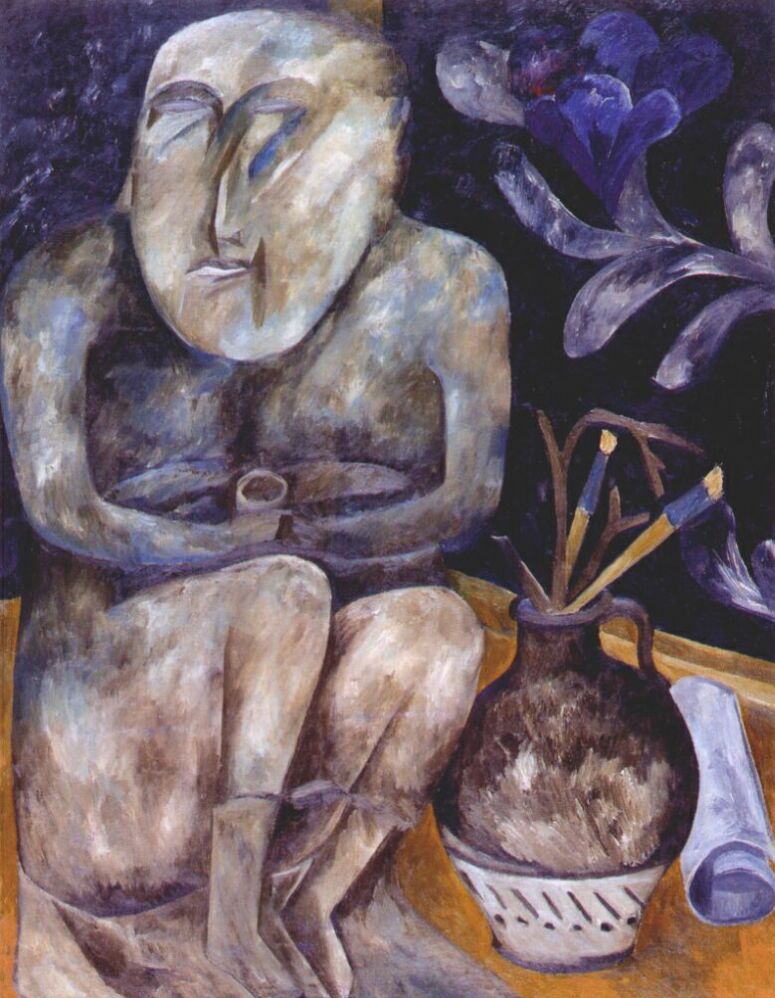The painting depicts a surreal, almost dreamlike scene featuring a heavyset, nude, and emaciated figure whose gender is difficult to discern. The figure, with an unusually large, elongated oval head comprising about a third of their torso, has hollow, sunken eyes and a vaguely forlorn or neutral expression. Their thin, emaciated arms wrap around their chest, while their thick legs are tucked up close to their torso and appear bound or restrained. The figure's skin ranges in color from gray to ashen blue and brown, and they sit slightly to the left on a light brown wooden surface. 

To the figure's right is a dark charcoal gray and white vase with black lines, filled with sticks or branches adorned with blue tips or strips of fabric. This vase also seems to hold three or four brushes. The background includes a dark wall with an abstract purple flower painted on it and a rolled-up parchment lying near the vase. Additionally, there are abstract branches and purple flowers painted around the scene, enhancing the surreal and expressionistic style of the artwork.